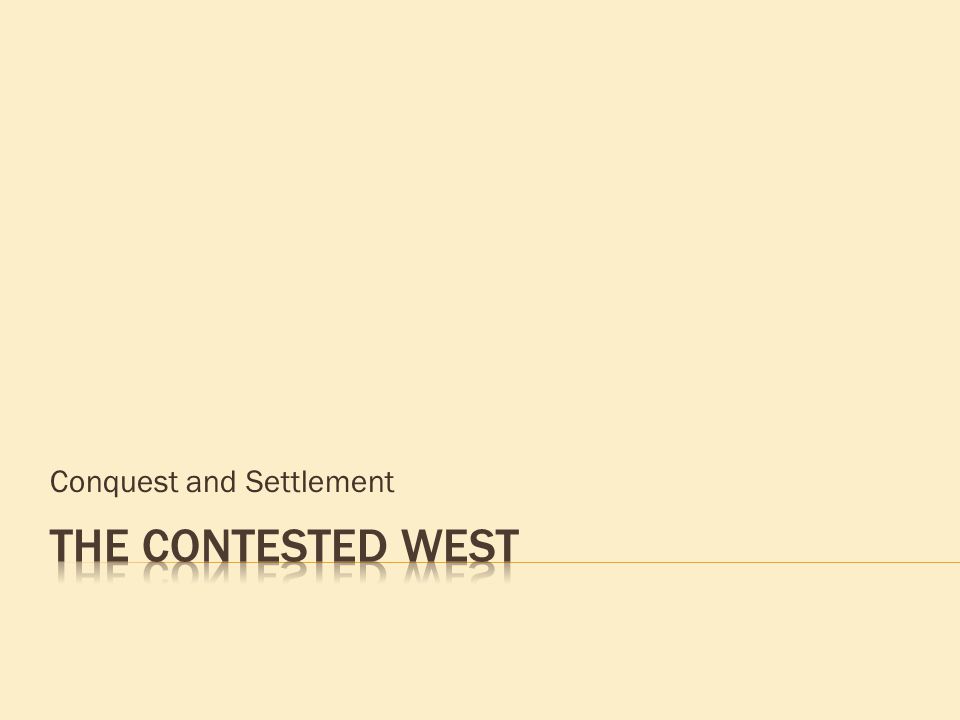This image features the title slide of a presentation, characterized by a minimalistic design and a light beige background. Dominating the bottom left corner, two lines of text sit against the creamy backdrop. The first line, "Conquest and Settlement," is typed in a regular brown font. Directly beneath it, in a larger, bold font with capitalized letters, it reads "THE CONTESTED WEST," accompanied by a subtle shadow that gives the text a reflective appearance. A very thin, yellow line runs horizontally from the left, starting at the word "THE," and extends to the right edge of the slide. The rest of the slide is empty, enhancing the stark contrast and simplicity of the design.